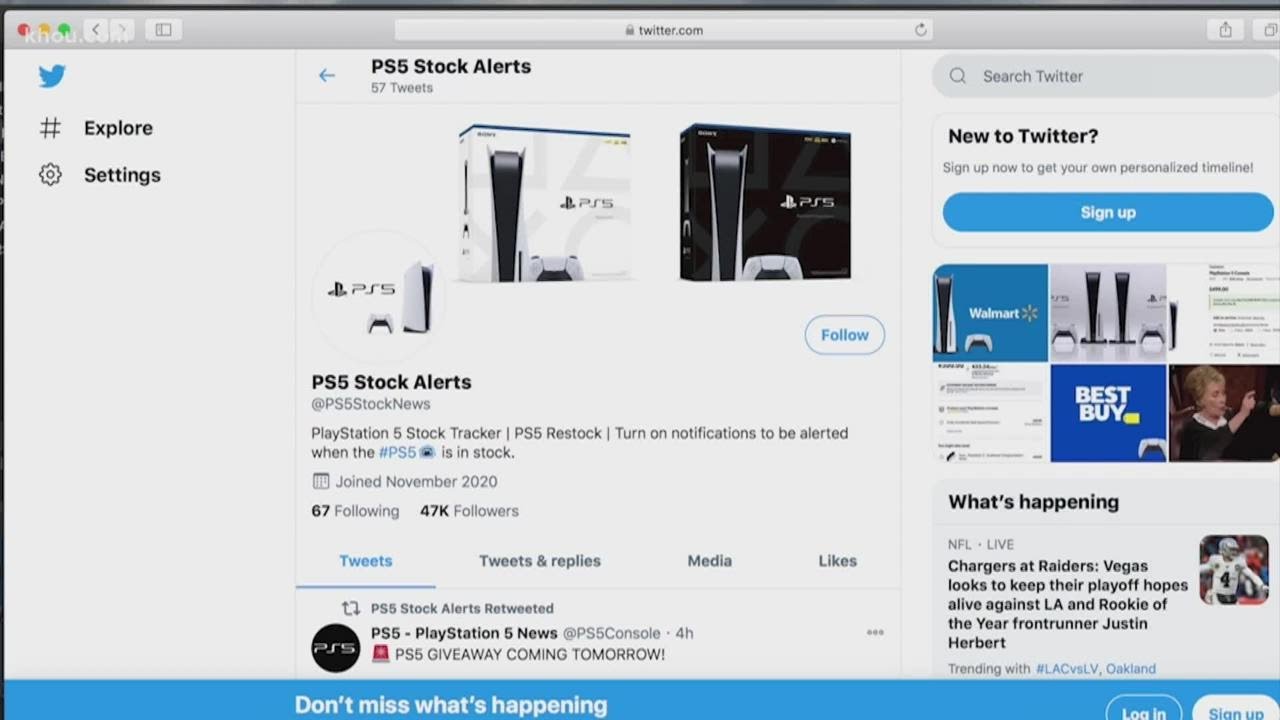The image depicts a Twitter webpage featuring a profile dedicated to PS5 stock alerts. At the top, a gray-colored bar spans across the page, with red, yellow, and green circles located in the upper left corner. The address bar centrally displays "twitter.com." Beneath it, the primary interface showcases a white background with the Twitter bird icon labeled as "Explore" and "Settings" in the upper left.

In the center of the page, the profile header reads "PS5 Stock Alerts," showing it has made 57 tweets. Below the header, there's an image of PlayStation 5 consoles, including one in its box and another standing upright outside the box. The left console is the disc-based version in a white box, while the right is the digital-only version in a black box. On the right side of the profile header, the "Follow" button is visible. The username "PS5 Stock News" is displayed below this button. The overall theme of the page reflects its sole purpose of informing users about the availability of PlayStation 5 consoles during a period when they were exceptionally scarce and difficult to obtain.